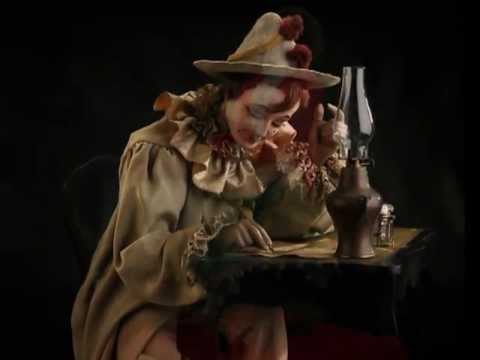In this evocative image, a figure is seated at a table shrouded in darkness, the background entirely black, which amplifies the subject's presence. The figure, possibly a sculpture, is dressed in an elaborate clown or joker costume of a beige, almost gold hue. A small witch-like hat adorned with burgundy furry balls sits atop their head. The figure's hair is a dark brown or reddish color, and their face is notably pale, enhanced with makeup that accents their slight blue eyes. 

The figure is focused on a piece of paper on the table, one hand resting on it while the other hovers in the air with two fingers almost touching, adding to the scene's enigmatic atmosphere. The costume includes frills at the end of the sleeves and a frilly, silky neckpiece, contributing to its theatrical appearance. The expression is subtle, with a faint smile. An oil lamp, modern in style but unlit, also adorns the table. The chair, barely distinguishable against the dark backdrop, is black, blending seamlessly with the surroundings. The entire setting and the sepia tone of the figure give the image a nostalgic, yet mysterious feel.